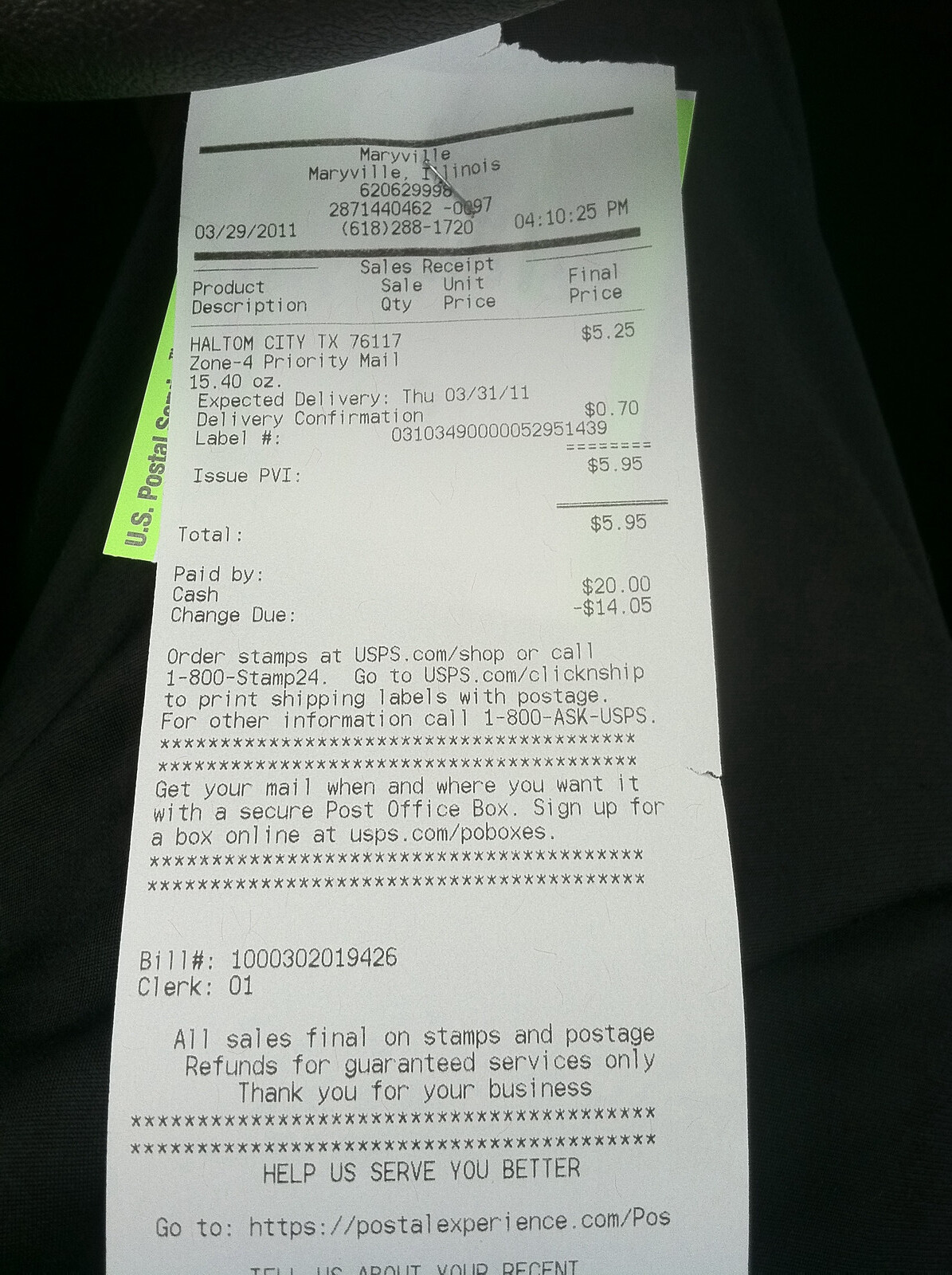A detailed photograph features a receipt stapled to a vivid, neon green sticker or label. The bright green sticker prominently displays "U.S. Postal Service" written in black. The white receipt layered in front was issued at the Maryville, Illinois post office on March 29, 2011, at precisely 4:10:25 p.m. The receipt includes the post office's contact number, 618-288-1720. It itemizes services purchased amounting to $5.25, $0.70, and a total of $5.95. Additional information on the receipt outlines services such as ordering stamps and applying for a post office box. The bill number and the clerk ID, which is 01, are also visible. This entire setup is placed against a black background that appears to be a textured black fabric, further enhancing the visibility of the receipt and sticker.